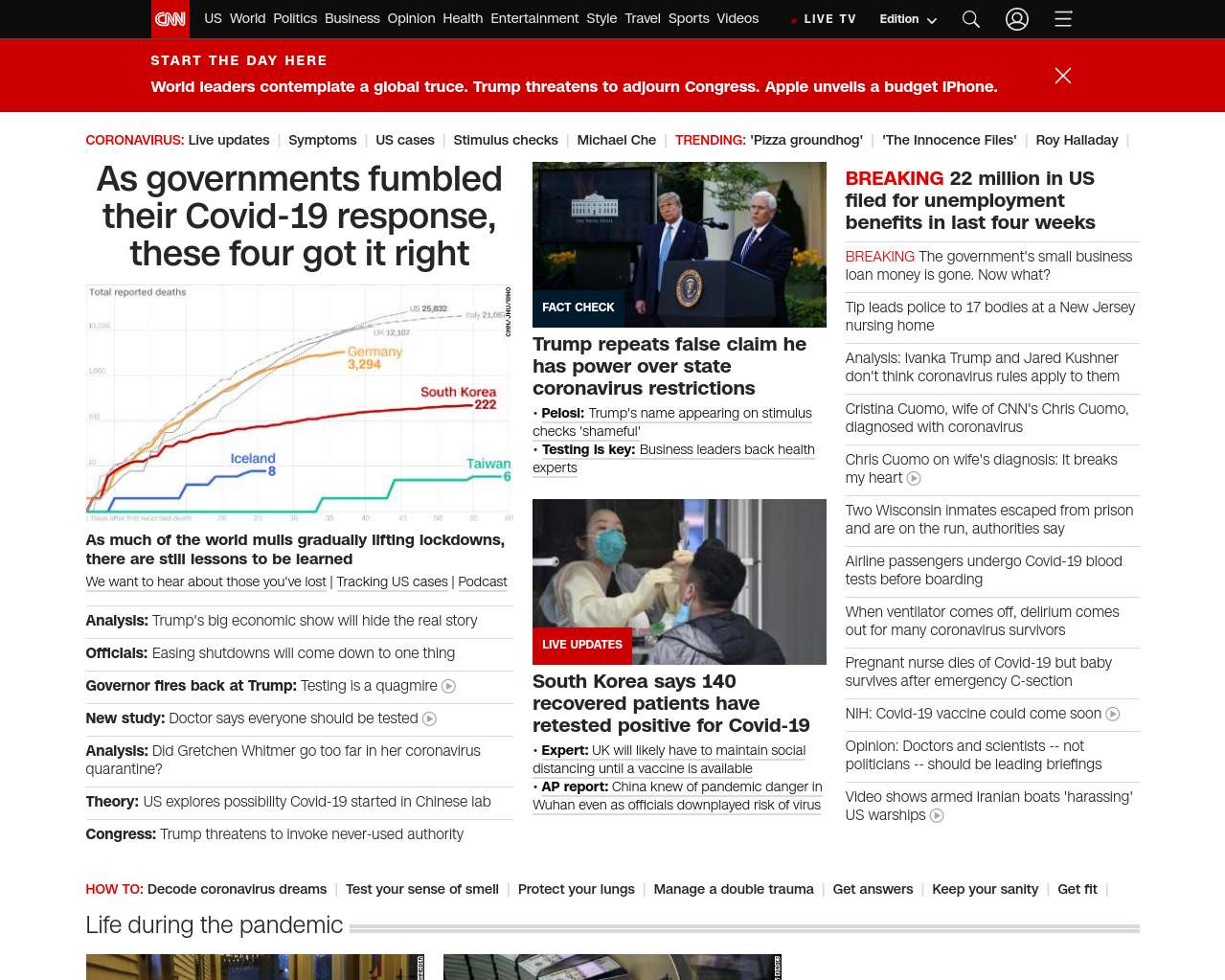This detailed caption provides an in-depth look at a CNN News web page, describing the layout and contents meticulously. 

---

**A Detailed Overview of CNN News Web Page**

At the top of the CNN News web page, various tabs are organized to provide easy navigation for users. These tabs include: U.S., World, Politics, Business, Opinion, Health, Entertainment, Style, Travel, Sports, and Videos. A red dot labeled 'Live TV' signifies real-time broadcasts, accompanied by an 'Edition' dropdown menu, a search box, a user icon, and a hamburger menu for additional options.

Highlighted prominently below the navigation tabs is a section titled "Start the Day Here," featuring major headlines: "World Leaders Contemplate a Global Truce," "Trump Threatens to Adjourn Congress," and "Apple Unveils a Budget iPhone." 

A secondary row of tabs follows focusing on more specific and trending topics: Coronavirus, Live Updates, Symptoms, U.S. Cases, Stimulus Checks, Michael Che, Trending, Pizza Groundhog, The Innocent Files, Roy Halladay.

The primary article on the page is titled "As Governments Fumbled Their COVID-19 Response, These Four Got It Right," illustrating successful pandemic responses from Iceland, Taiwan, South Korea, and Germany with an accompanying graph.

To the right of this article is a photograph featuring former President Donald Trump and Vice President Mike Pence standing at a podium. Embedded within the photograph is a 'Fact Check' label. The caption beneath this image reads, "Trump Repeats False Claim He Has Power Over State Coronavirus Restrictions."

Below, another image depicts a woman wearing a surgical mask swabbing the face of a man in a jacket. The photograph is tagged with 'Live Updates,' and the article caption states, "South Korea Says 140 Recovered Patients Have Retested Positive for COVID-19."

On the right side of the page, a breaking news banner announces, "$22 Million in U.S. File for Unemployment Benefits in the Last Four Weeks," emphasizing the economic impact of the pandemic.

---

This complete description provides a thorough visual and contextual overview of the CNN News web page, making it easy to visualize the layout and key content highlights.